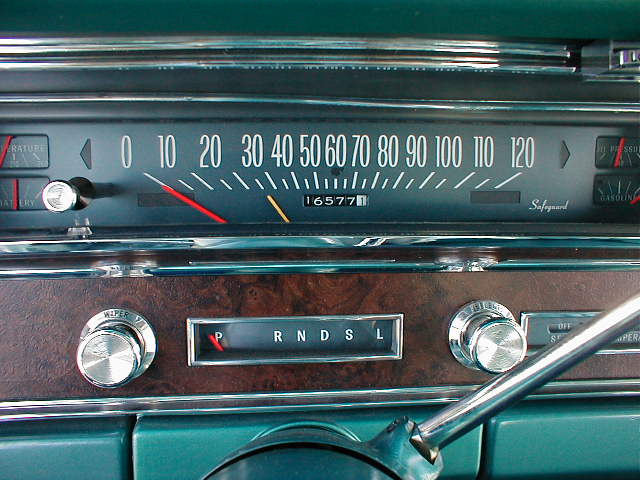The image depicts the dashboard of a classic family automobile from the 1960s or 1970s. Central to the dashboard is a stationary speedometer, featuring white-painted numerals that span from 0 to 120 miles per hour. The speedometer is decidedly analog, devoid of any digital elements. Below the speedometer, a signature reads "Safeguard." The mileage indicator on the speedometer shows 16,577.1 miles. Below this central gauge sits a radio set against a faux wood panel. The radio has two primary controls: a volume knob on the left and a tuning knob on the right. Positioned lower on the dashboard, connected to the steering column, is the shifter knob, with an adjacent parking and gear indicator set to park. The gear options labeled next to it include RNDSL, standing for Reverse, Neutral, Drive, Standard, and Low transmission settings. This detailed dashboard exemplifies the vintage design and craftsmanship typical of automobiles from that era.